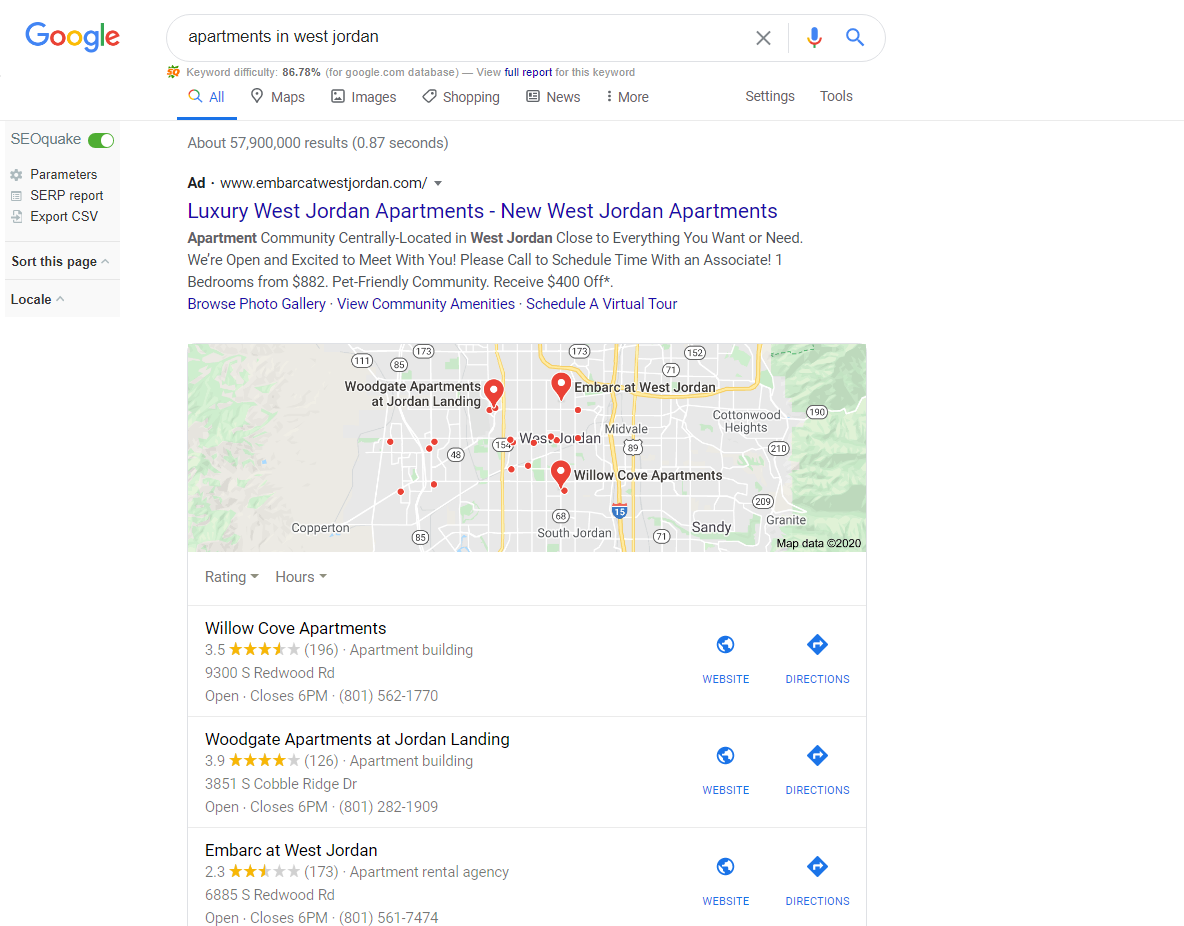**Detailed Descriptive Caption:**

The image showcases the results of a Google search for "apartments in West Jordan". In the upper left-hand corner, the iconic Google logo and the search bar are visible, confirming the platform used for the search. Adjacent to it is an active SEOquake plugin indicated by a green oval with a white toggle button. Below the SEOquake section, options such as parameters, SERP report, export, CSV, sort this page, and locale are listed.

Dominating the page is the primary search result area, starting with a metric showing the keyword difficulty at 86.78% for the Google.com database, with an option to view the full report. The search categories are arranged horizontally beneath the search bar, including All, Maps, Images, Shopping, News, More, Settings, and Tools, with "All" being highlighted in blue.

The search yielded approximately 57,900 million results in 0.87 seconds. The top result is an advertisement for "Embark at West Jordan", promoting luxury and new apartments centrally located in West Jordan. It emphasizes their excitement to welcome prospective tenants and offers a starting price of $882 for one-bedroom apartments, mentioning a pet-friendly policy and a $400 discount. There are additional hyperlinks to browse the photo gallery, view community amenities, and schedule a virtual tour.

Below the ad, a Google map displays locations related to the three listed apartment results, indicating map data from 2020. The three highlighted apartment listings are:

1. **Willcove Apartments**:
   - Rating: 3.5 stars from 196 reviews.
   - Description: Apartment building.
   - Address: 9300 South Redwood Road.
   - Operation Hours: Open, closes at 6 p.m.
   - Phone: 801-562-1770.
   - Hyperlinks: Website, Directions.

2. **Woodgate Apartments at Jordan Landing**:
   - Rating: 3.9 stars from 126 reviews.
   - Description: Apartment building.
   - Address: 3851 South Cobble Ridge Drive.
   - Operation Hours: Open, closes at 6 p.m.
   - Phone: 801-282-1909.
   - Hyperlinks: Website, Directions.

3. **Embark at West Jordan**:
   - Rating: 2.3 stars from 173 reviews.
   - Description: Apartment rental agency.
   - Address: 6885 South Redwood Road.
   - Operation Hours: Open, closes at 6 p.m.
   - Phone: 801-561-7474.
   - Hyperlinks: Website, Directions.